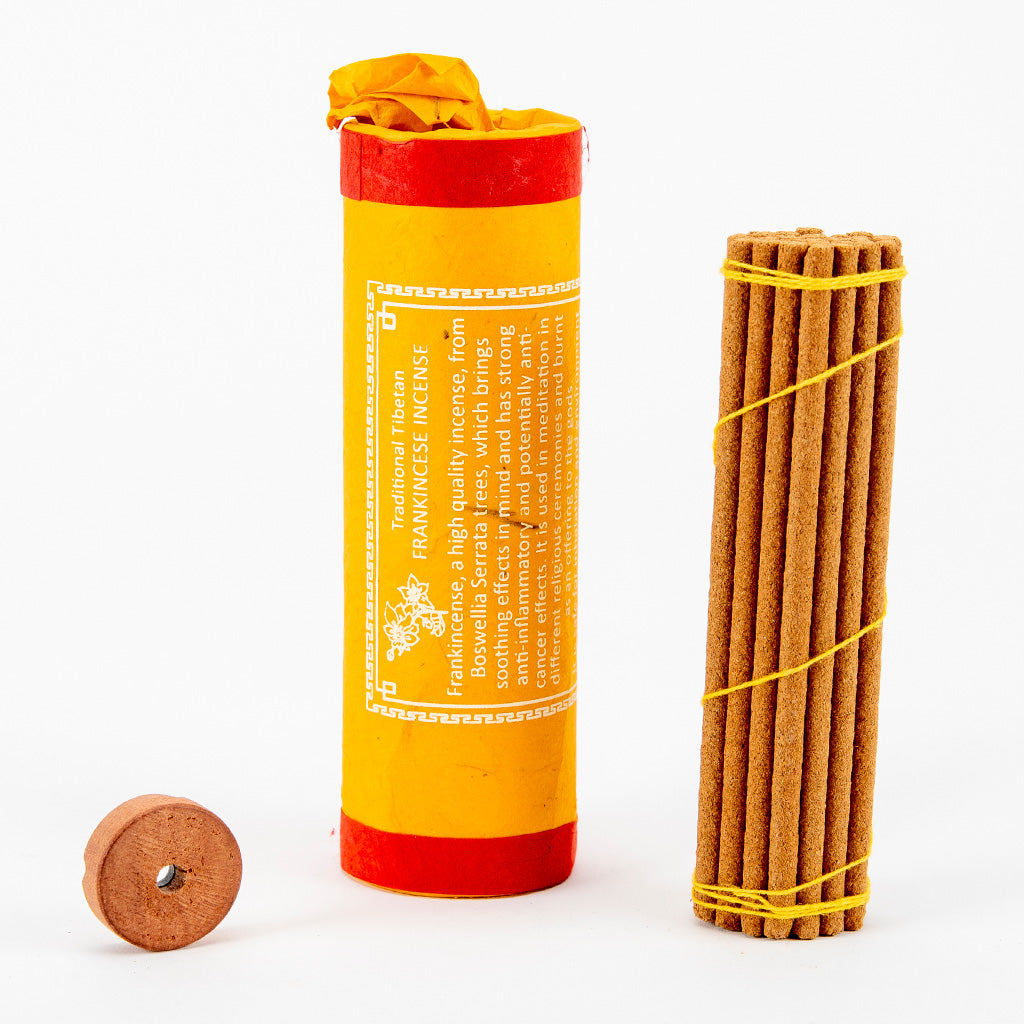The image showcases packaging and sticks of traditional Tibetan frankincense incense against a white background. The cylindrical canister is predominantly marigold yellow with red banners at the top and bottom, boasting white lettering that reads, "Traditional Tibetan Frankincense Incense." The detailed description on the package highlights that frankincense, derived from Boswellia cerata trees, is renowned for its high quality and soothing effects on the mind, as well as its strong anti-inflammatory and potential anti-cancer properties when used in meditation. Adjacent to the canister are approximately 20 brown incense sticks, bundled together with a marigold cord. A small circular incense holder, designed with a hole for holding and burning the incense, is visible to the left of the canister.